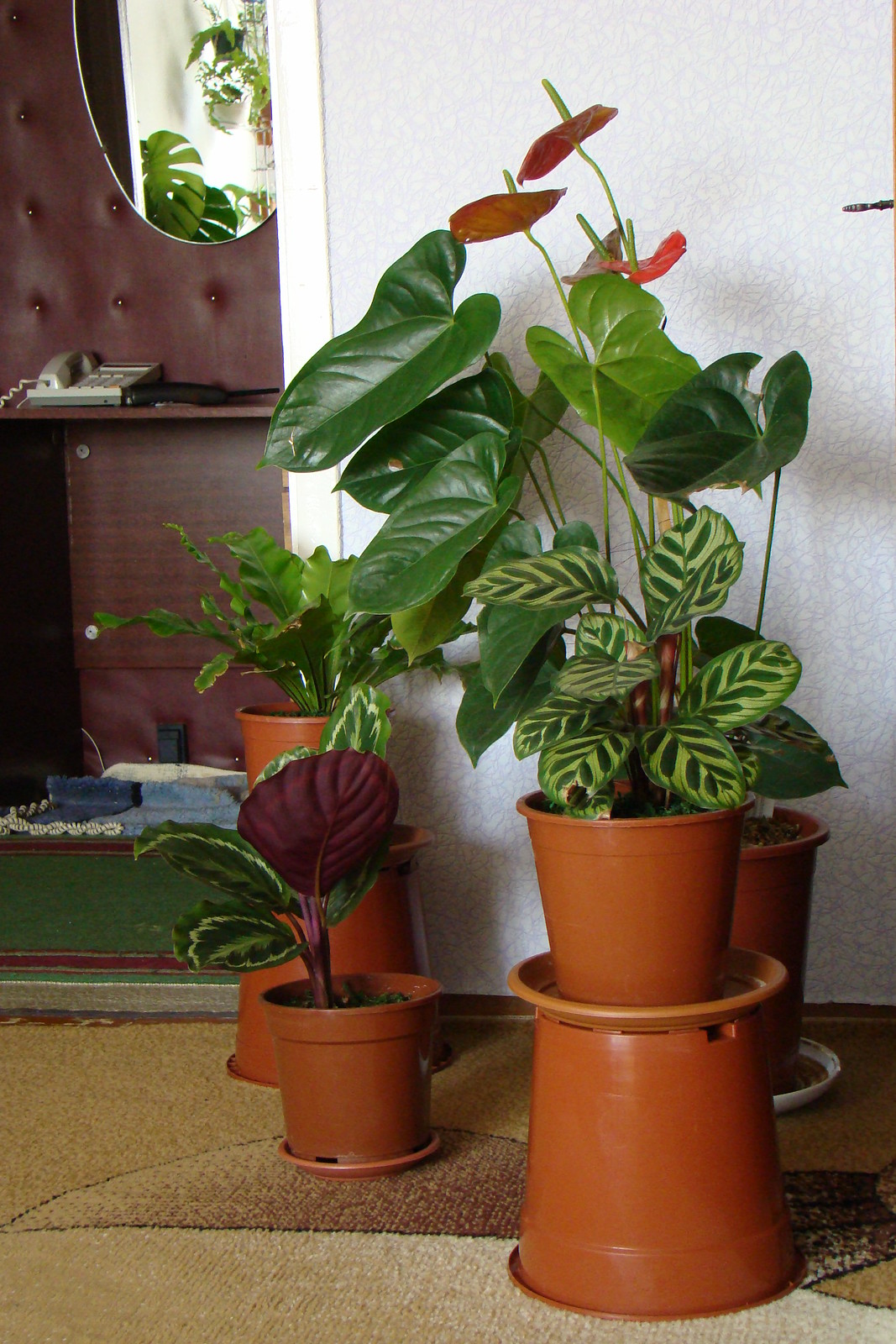This photograph showcases a beautifully arranged indoor garden, highlighting the care and dedication of an enthusiastic plant lover. The focal point features a terracotta-colored plastic pot sitting atop a larger inverted pot, with dark green leaves featuring light green feathering emerging gracefully, resembling feathers. The arrangement includes various plants, some sporting broad lily pad-like fronds and flat, red flowers with distinctive green stems. The plants rest on a carpet that transitions from light to dark brown, accented by patches of white. On the left wall, an open door reveals a burgundy room with a green carpet, and a telephone on a desk. Adjacent to the door, a mirror reflects more greenery, enhancing the sense of abundance. To the right, there's a dark brown laminated wood wall, complemented by a dark brown leather wall featuring a mounted phone and a green shelf with red lining below it. The background wall, adorned with off-white wallpaper, further frames this lush indoor sanctuary.